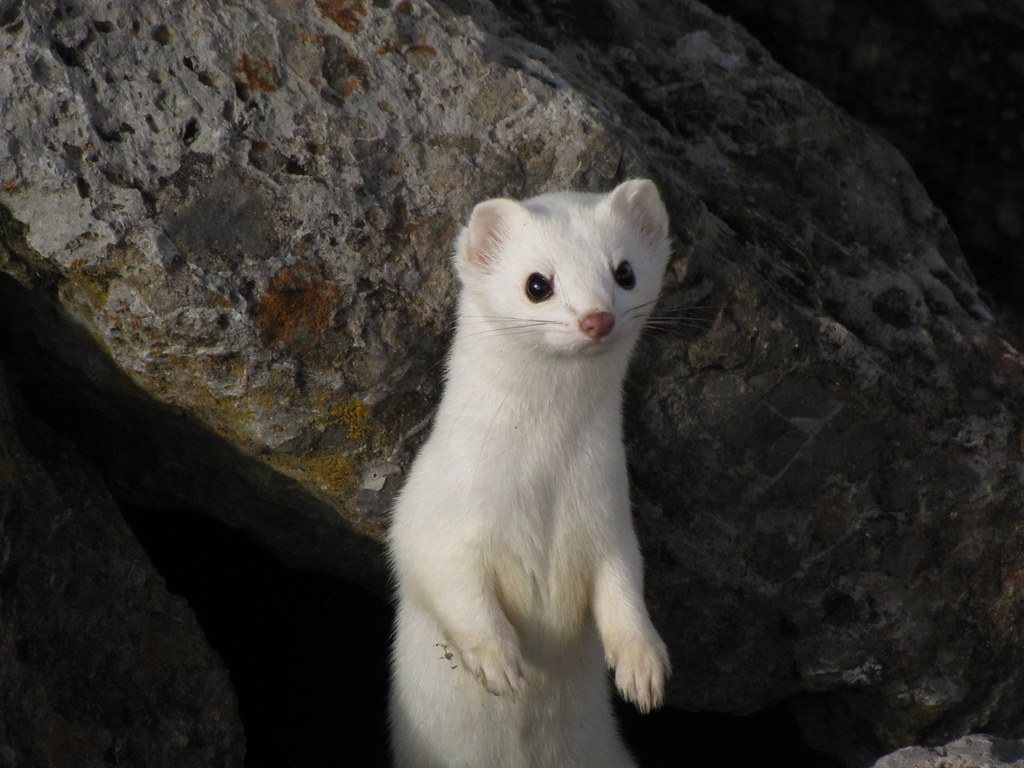An up-close photo captures a curious, white-furred member of the mustelid family, possibly a mink or weasel, standing upright on its hind legs. The small creature's delicate paws are held slightly forward, displaying its alert posture. It has large, expressive black eyes, a charming red nose, and multiple black whiskers that extend from its face. Slightly pinkish ears complement its endearing appearance. This scene is set against a backdrop of a large, dark gray and black rock, tinged with hints of red and green, potentially indicating moss or some form of growth. The rock appears significant in size, towering over the petite animal. The image, likely taken outdoors in dim lighting, accentuates the inquisitive nature of the creature as it seems to be observing something intently.